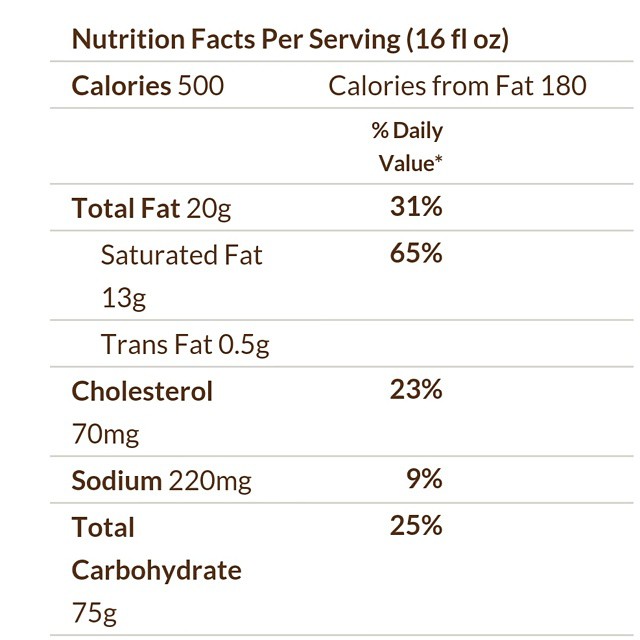The image captures a detailed table of nutritional facts per serving, clearly marked for a serving size of 16 fluid ounces. The table is bordered and divided by gray lines, which neatly separate each category for readability. The text, formatted in dark brown, lists the following values: 500 calories, with 180 of these calories coming from fat. The rightmost column details the percentage of daily values: 20 grams of total fat equates to 31%, of which saturated fat is 13 grams (65%) and trans fat is 0.5 grams. Cholesterol amounts to 70 milligrams (23%), sodium is 220 milligrams (9%), and total carbohydrates are 75 grams (25%). The layout suggests it could be from the back of a food container, though no specific food item or packaging is visible in the image. This detailed breakdown would be particularly useful for individuals managing their dietary intake or those on specialized diets.